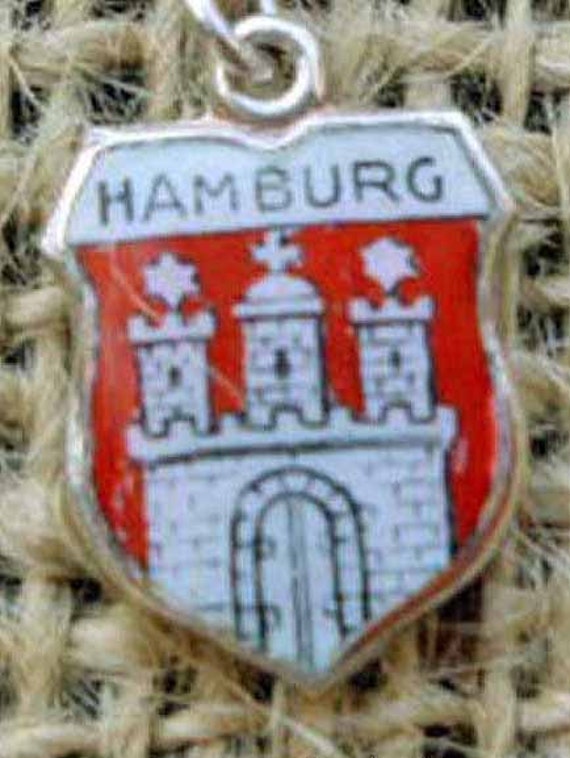The image features a silver-edged badge, shaped like a seal with a slightly pointy base, attached to a hand-wrapped, cross-weaved hemp surface. The top of the badge has a loop for attachment, making it versatile as a brooch, keychain, or pin. At the top of the badge, the word "Hamburg" is printed in black capital letters on a white background. Below the text is a red background showcasing a detailed, hand-drawn white castle. The castle features a large arched entrance flanked by three tall towers; the left tower is topped with a star, the middle with a cross, and the right with another star. Each tower also has a window. The badge overall resembles a decorative crest, possibly German in origin, and exudes a sense of jewelry or pendant craftsmanship, with a slight tilt to the left enhancing its intricate presentation.